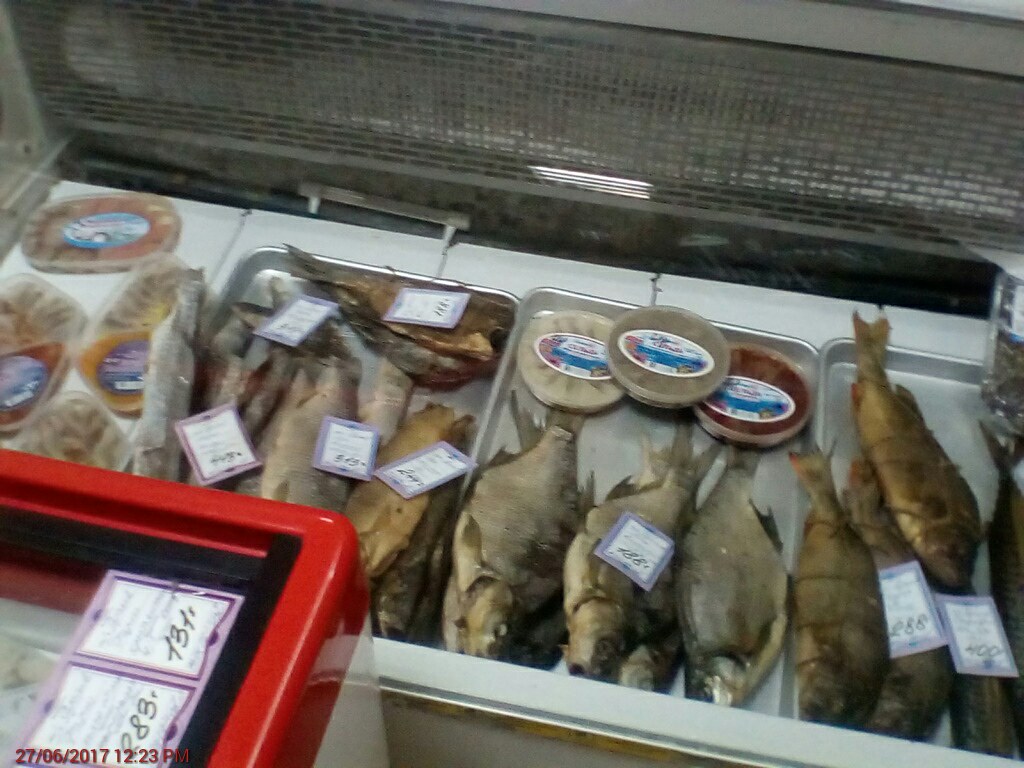In this detailed image, a white freezer or display case with its lid open reveals an array of various seafood items neatly organized in trays. The focal point is three silver trays filled with freshly caught, unwrapped fish in shades of brown and gray. Each fish is marked with price tags, suggesting they are for sale, likely in a market or store. Among the fish, small containers with labeled contents, possibly dips or other seafood products, are nestled within the trays. 

On the left side of the display, there are individually wrapped packages, potentially containing ham steaks or salmon steaks, each with visible labels, though the exact details are indistinguishable. Behind the fish trays, a black grill indicates an element of the cooling system, which might close to maintain the chilled environment. In the bottom right-hand corner, another part of the freezer is visible, with some labels that are unclear. Additionally, the left corner of the image features a red frame with white labels bordered in purple, inscribed with black writing, though the specifics are not legible. The photograph vividly captures the setup of a typical seafood market display, showcasing both the fish and accompanying food items under market lighting.